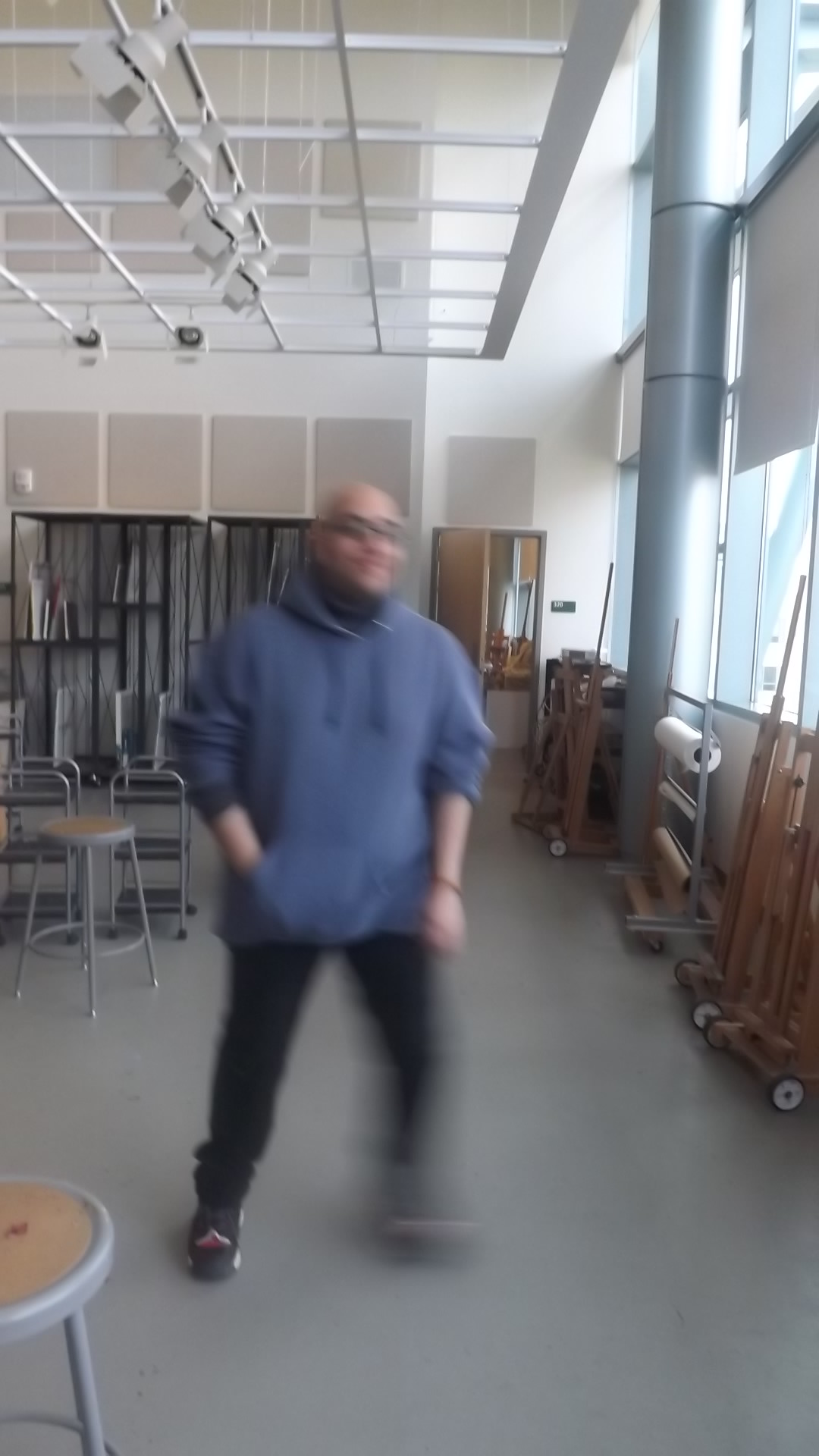The image depicts a bald man with a blue pullover hoodie sweatshirt, black pants, and black shoes featuring a red triangle on the front, standing in what appears to be an art studio or art classroom. His thick red glasses and entire right side, including his face, are blurred, suggesting movement. The background is clear and detailed, showing black shelves with art canvases and paint easels. Additional elements include a wooden stool with a gray rim in the foreground, upside-down stools, various chairs, and stools on wheels scattered around the room. Overhead, bright white stage lights are set in a metal grid. A large silver pole and windows on the right side of the room, allowing natural light to come in, further establish the setting as a spacious, well-lit studio or classroom.